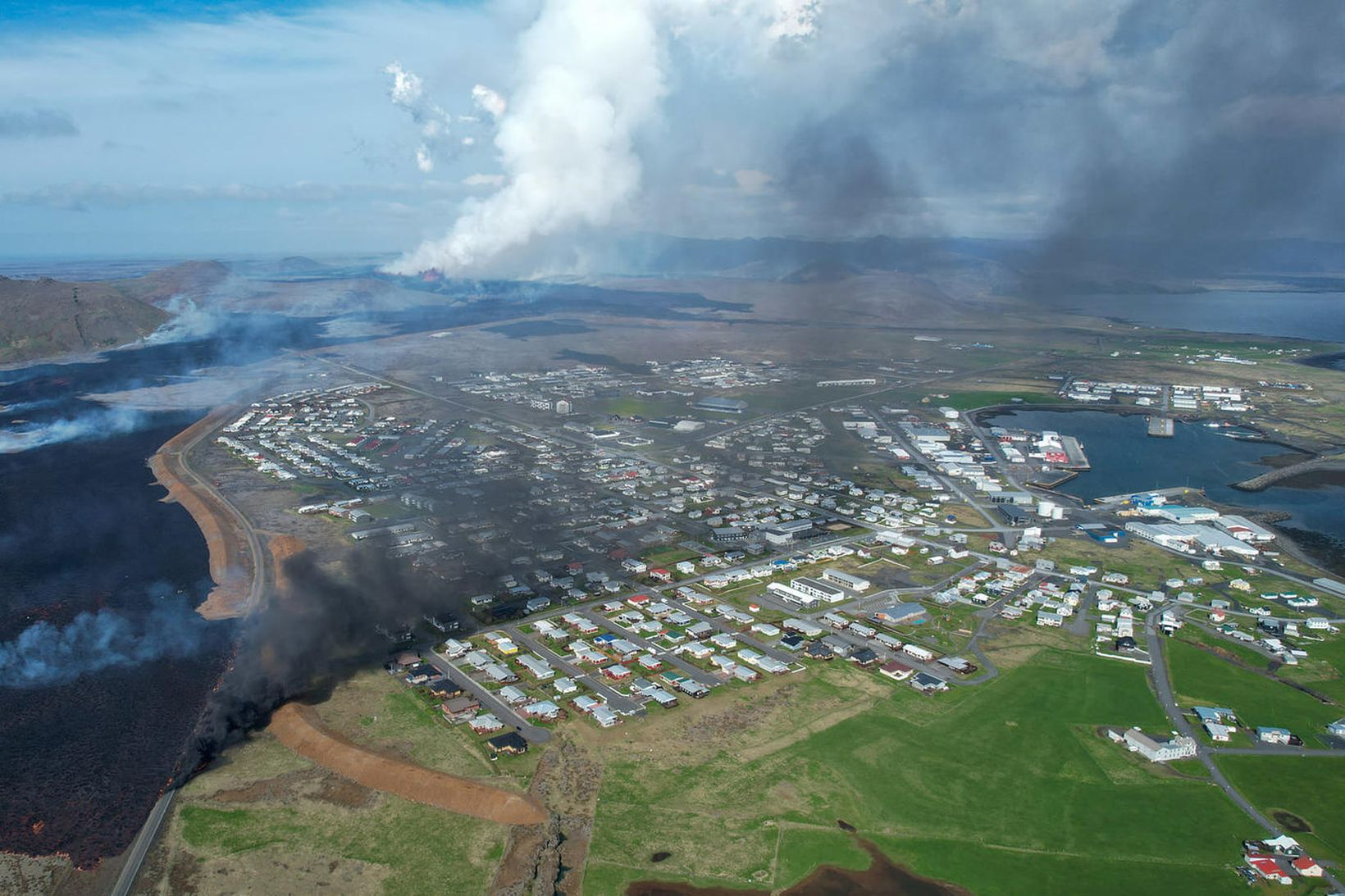This aerial photograph captures a dramatic contrast between serene residential life and the raw power of nature. In the foreground, neatly arranged clusters of white and light-colored houses are set amidst patches of green lawns and well-planned streets, epitomizing a peaceful, orderly suburban landscape. On the left side of the image, however, the scene starkly shifts as a vast expanse of black lava slices through the town. The sharp, dark edge of the lava flow cuts across roads and disrupts the otherwise tranquil environment, evidence of its destructive path. Amidst the residential zones, clusters of industrial and commercial buildings can be seen, interconnected by a network of roads branching out across the town. Further in the background looms the source of this disruption: a massive plume of white smoke billowing from the volcanic eruption, merging dramatically with the clouds above. This powerful image poignantly illustrates the fragility of human settlements in the face of nature’s overwhelming force.